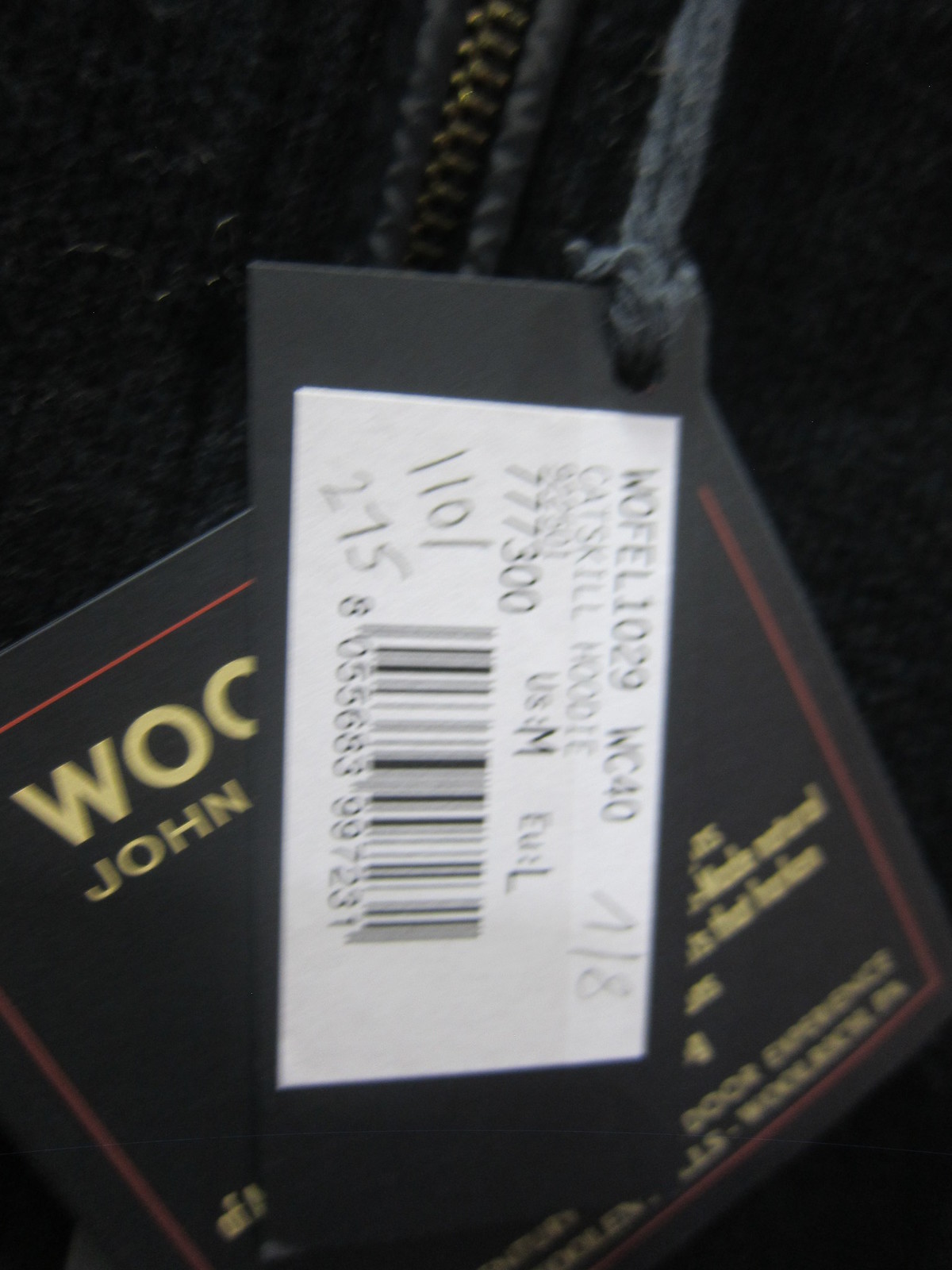This is a photo showcasing the price tag and designer tag attached to a piece of fuzzy clothing. A striking gold zipper runs up the back of the garment. The tags are secured with a black piece of yarn. There are two distinct tags, both black. The one in the background features the letters "W-O-O" written in gold, bordered by a red line, and includes the word "John" along with other text stating "a door experience." The tag on top, which appears to be the price tag, contains a barcode and some handwritten numbers.